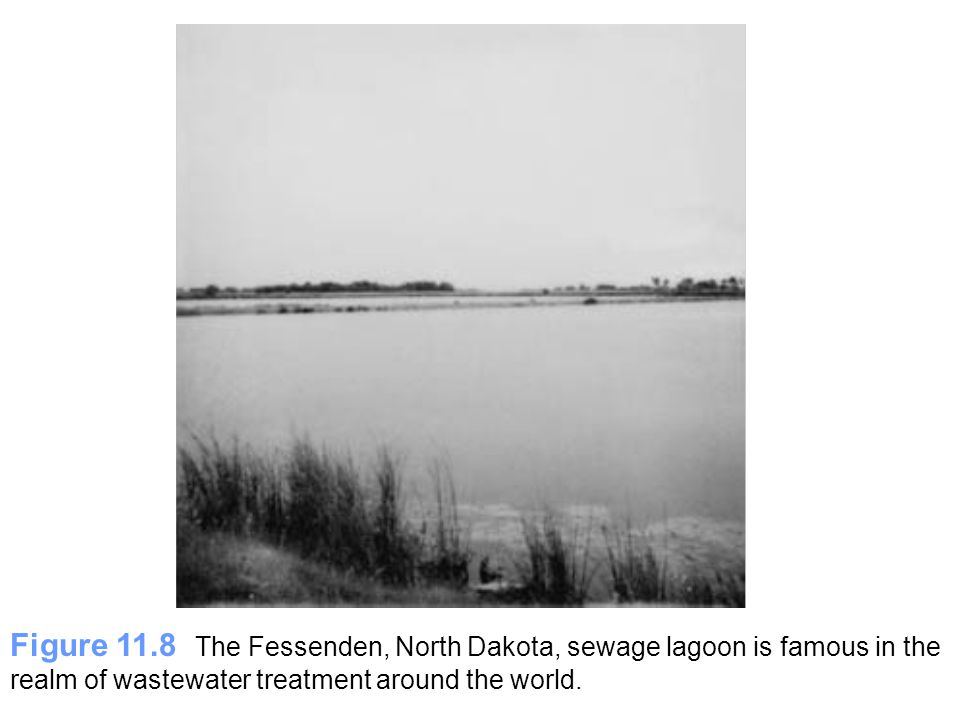This black and white photograph, labeled "Figure 11.18," showcases the renowned Fessenden, North Dakota Sewage Lagoon, esteemed globally for its contributions to wastewater treatment. The expansive lake is surrounded by dry brush and shrubbery, with noticeable green plant life, including weeds sprouting along the shoreline. Interestingly, the lake appears bisected by a slender land bridge, scarcely three feet wide. A frothy foam is visible at the water's bottom, and in the bottom right corner, the water seems to swell. Intriguingly, a man's face can be faintly discerned within the depths of the water. Though the overcast ambiance of the gray day is muted by the monochrome palette, the stark contrasts add depth and texture to this intriguing image.